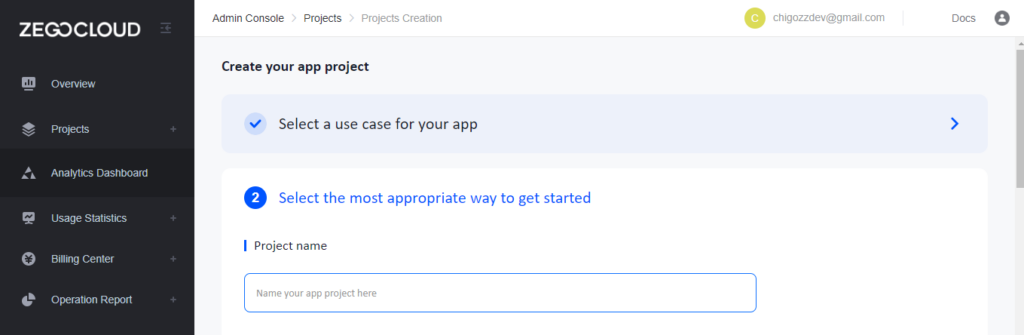This screenshot displays the ZegoCloud website interface, predominantly featuring a white background. On the left-hand side, there is a black vertical column with the large white text "ZEGOCloud." Beneath this header, a menu lists different sections, each accompanied by a distinct icon. The first icon resembles a television and is labeled "Overview." Next, an icon resembling a stack of papers represents "Projects." Following this is a triangle icon with another triangle inside it, labeled "Analytics Dashboard." A computer monitor icon signifies "Usage Statistics." Additionally, a circle icon with a Y and two lines through it is labeled "Billing Center," and lastly, a Pac-Man-like circle icon with a missing pie slice denotes "Operation Report."

In the center of the screen, the header line reads "Admin Console" with a right arrow, followed by "Grade Out Projects" and another right arrow leading to "Grade Out Projects Creation." Below this navigation trail, the main heading in bold letters states "Create Your App Project." Adjacent to this title is a blue circle containing a checkmark, accompanied by the instruction "Select a Use Case for Your App." Below, another section begins with a blue circle marked with the number two, directing users to "Select the Most Appropriate Way to Get Started."